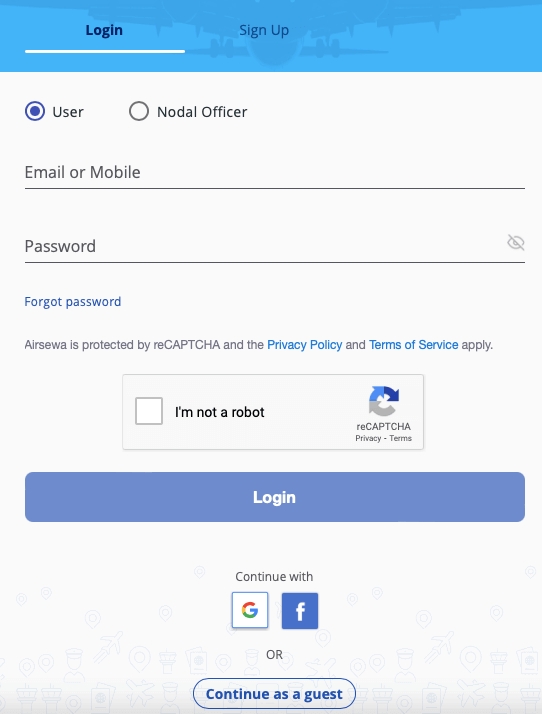The image features a blue rectangular tile with options to either "Log In" or "Sign Up." It displays fields for the user to enter their email or mobile number and password, with an option to view the password by making it visible if desired. Additionally, there is a "Forgot Password" link available. The form is secured by reCAPTCHA, featuring a checkbox for "I'm not a robot," along with links to the privacy policy and terms of service. Options to "Log In" and "Continue" are prominently displayed, with alternative login methods through Facebook and an option to "Continue as a Guest." The background is white, and various icons are subtly integrated in the backdrop.